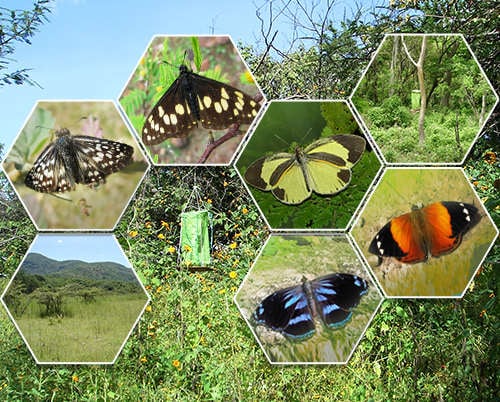In the photograph, a vibrant outdoor scene serves as the backdrop, featuring a lush, green hill adorned with numerous yellow wildflowers beneath a clear blue sky. Central to the image, a green fabric bag or bird feeder hangs from a tree, further adding to the natural ambiance. Superimposed over this picturesque landscape are seven hexagonal insets arranged in a honeycomb pattern. 

Each hexagon contains a distinct image, primarily showcasing different butterflies native to this habitat. The top-left hexagon displays a brown butterfly with yellow spots, while beside it is a butterfly predominantly yellow with brown-tipped wings and a long brown line. Adjacent to these is an enchanting black butterfly with vibrant blue patterns on its wings. 

Continuing clockwise, there's an orange butterfly with black-edged wings, adorned with three white spots. Another hexagon features a black butterfly with light yellow speckles. Lastly, there's a butterfly mostly yellow with black tips. Interspersed among these butterfly images are a couple of hexagons showing the natural surroundings: a grassy meadow with rolling hills and a part of the forest, adding depth and context to the scene. This detailed composition beautifully encapsulates the diversity and richness of the habitat.